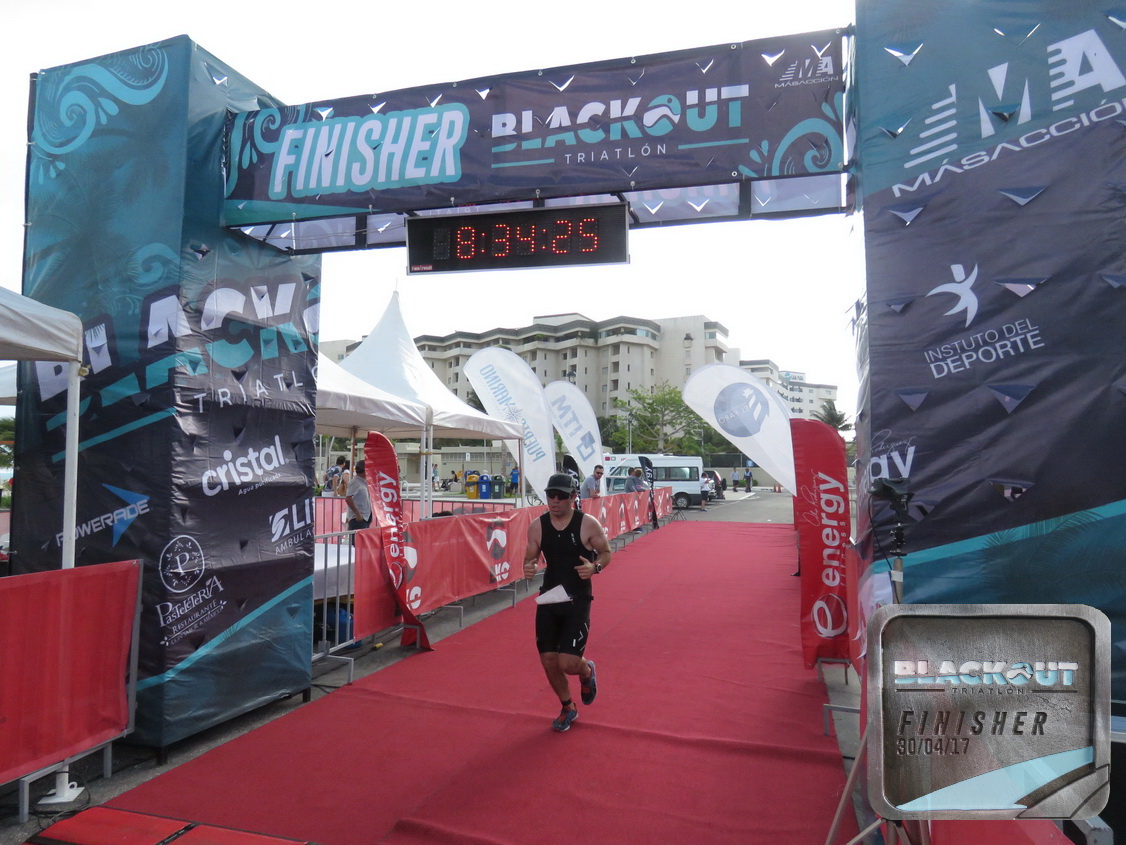The image depicts a person crossing the finish line of a race, possibly a marathon, with a recorded time of 8 hours, 34 minutes, and 25 seconds. The finish line is marked by an archway with green and black plastic tones, inscribed with "Finisher Blackout Triathlon." Banners are placed prominently at the top and on both sides of the arch, contributing to the celebratory atmosphere. Below, a timer displays the finishing time. The background reveals a big block of cream-colored buildings, while barricades wrapped in red plastic flank the sides of the red carpeted path the runner is traversing. Onlookers can see multiple energy stations and several tents nearby, presumably for participants' use. The bottom corner of the image reads "Blackout Finisher," along with the date "30-4-17," likely referring to April 30th, 2017.